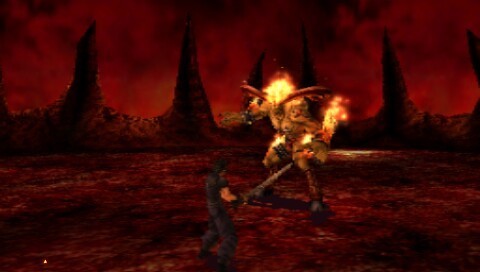A blurry screenshot captures a moment in a video game, depicting a dramatic scene filled with action and otherworldly elements. In the background, an ominous orange glow illuminates the horizon, highlighting five to six towering, jagged peaks reminiscent of menacing mountains, with significant gaps between them. The ground within the scene simmers like a volcanic wasteland, glowing an intense orange-red with blackened patches resembling lava pools. Dominating the middle of the screen is a monstrous creature, its body ablaze in a yellowish-golden hue. The beast stands on massive legs with gray feet and sports large, reddish horns, enhancing its fearsome appearance. In the forefront, a lone human figure clad in black attire contrasts sharply against the fiery backdrop. The character's white arms and elongated sword or saber suggest readiness for combat, poised to face the towering behemoth that looms above, more than twice the person’s height.